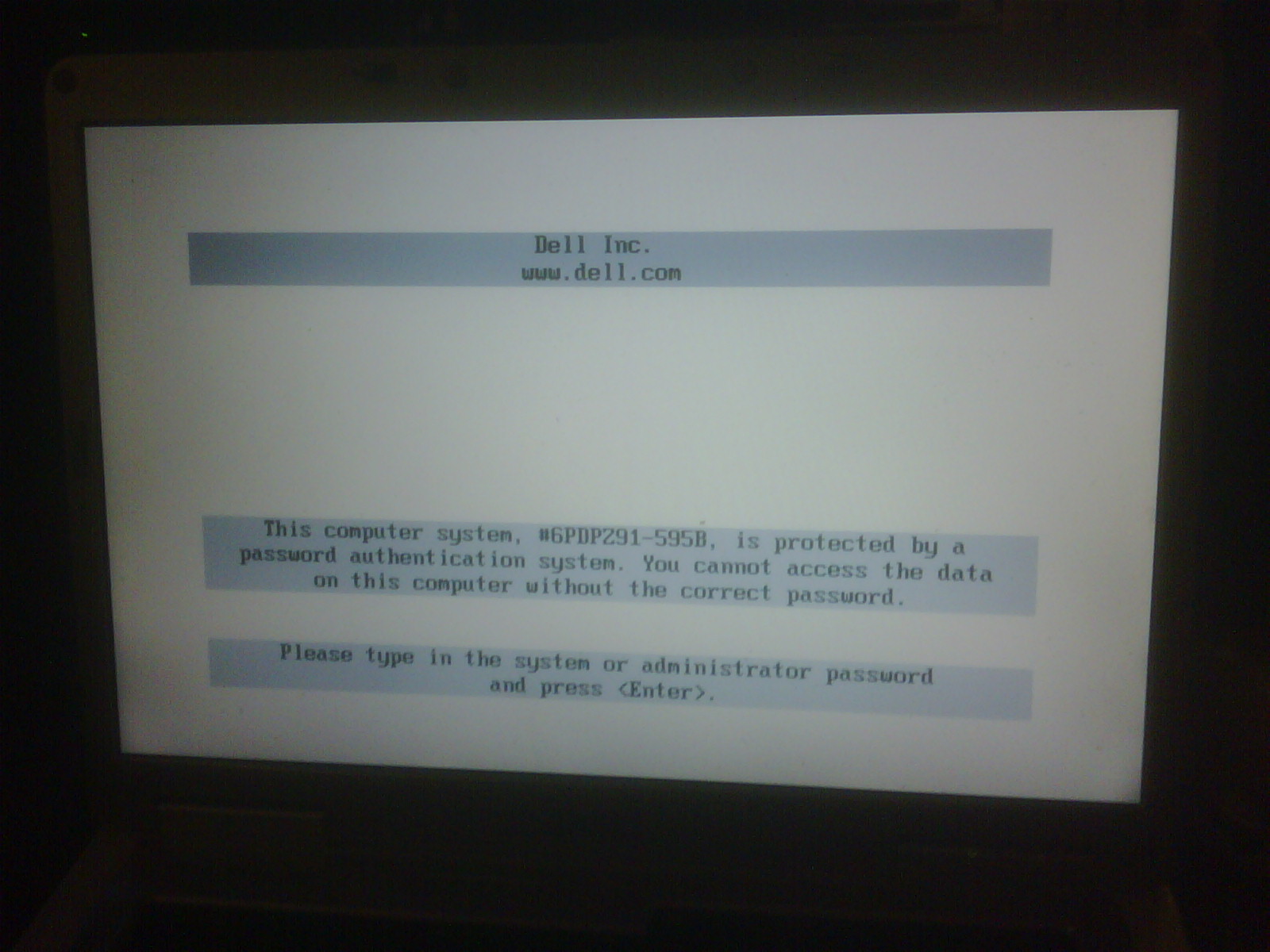The photograph depicts a slightly blurry and grainy image of a computer screen taken in a dark room, possibly using an old or low-quality camera. The screen itself, which is the only source of light in the image, appears slightly tilted from the lower left to the upper right. The background outside the screen is dark, and a faint light gray outline of the monitor and keyboard is barely visible.

The computer screen displays three horizontal blue rectangles with black text against a white background. At the top of the screen, the first blue rectangle contains the text "Dell Inc www.dell.com." Below this, with a significant gap of white space, the second blue rectangle reads, "This computer system number 6PDP291-595B is protected by a password authentication system. You cannot access the data on this computer without the correct password." The third and final blue rectangle instructs, "Please type in the system or administrator password and press enter." This setup suggests that the computer is in the process of booting up and awaiting a password to proceed.